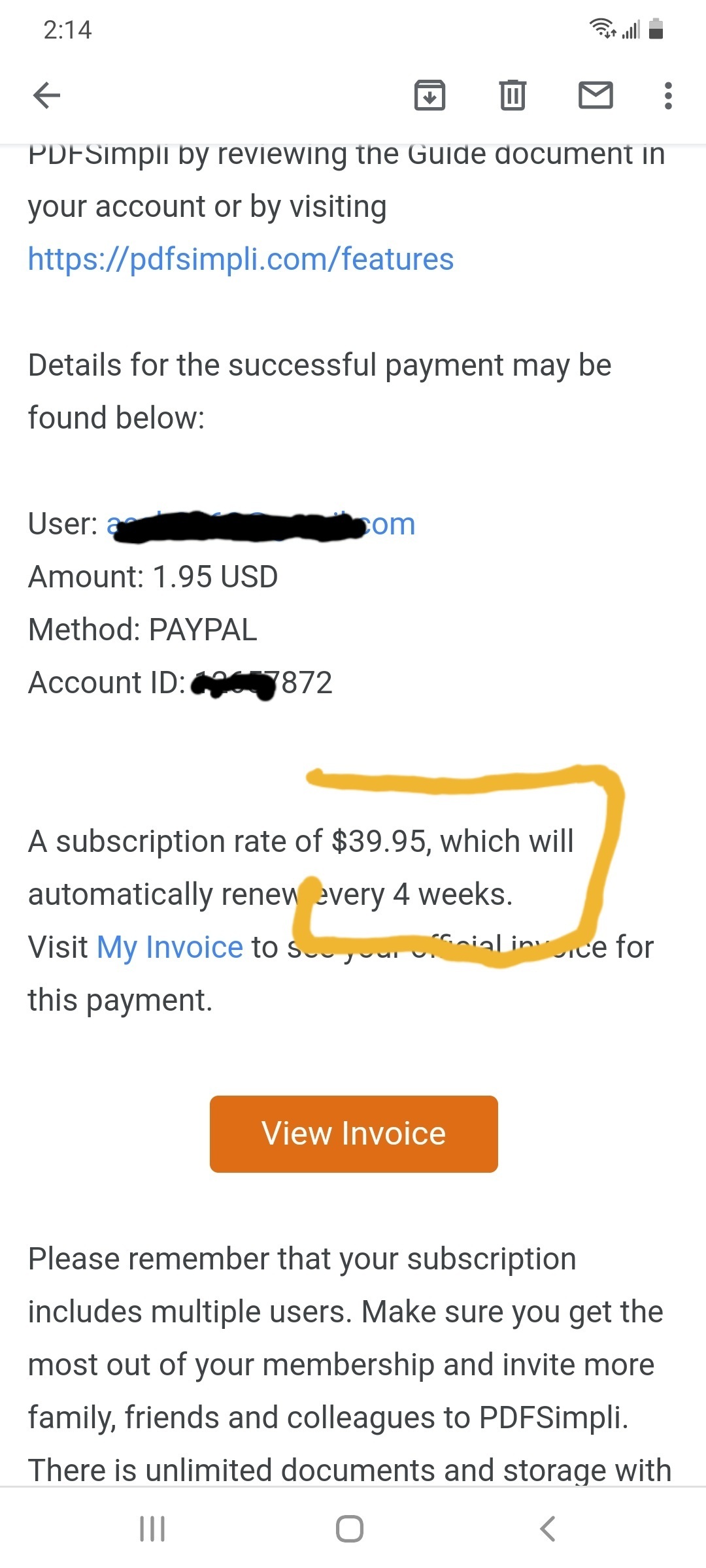Screenshot of a smartphone display showing details of a payment confirmation email from PDFSimply. The top of the screenshot indicates the time, Wi-Fi connection, signal bars, and battery percentage, revealing that it was taken from a smartphone. 

The email content features the following details:
- **PDFSimply** heading and a directive to review the guide document within the user's account or by visiting PDFSimply.com/features, with the URL highlighted in blue, suggesting it is clickable.
- A confirmation section that states, "Details for the successful payment may be found below," listing the user details, the payment amount of $1.95, and the payment method, which is PayPal. The account ID is also provided.
- A subscription information box indicating a recurring subscription rate of $39.95 that will renew every four weeks, with a prompt to visit 'My Invoice' to view the official invoice for the payment. An orange "View Invoice" button is included.
- A reminder that the subscription includes multiple users and encourages the user to invite family, friends, and colleagues to maximize the benefits of the subscription, which includes unlimited documents and storage.
- The email appears to cut off at the bottom, but it shows navigation buttons that are likely used to change screens.

The background of the email is white with black text, making the content clear and readable.